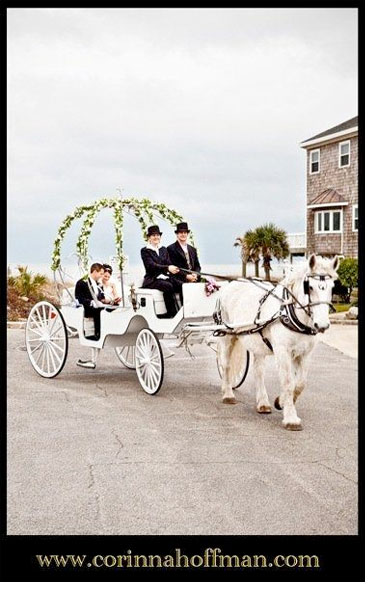The photograph captures a picturesque white horse-drawn carriage adorned with greenery and flowers arching over the top, gliding from left to right. The white horse leads the way, elegantly tethered to the ornate carriage featuring white wheels. Seated in the front, dressed in tuxedos with black top hats, are two individuals—likely a man and a woman—steering the horse. In the rear, a bride and groom are seated together, holding each other tenderly amid the floral decorations. The background reveals a scene of open sea or beach extending to the horizon on the left, contrasted with a stone brick building to the right. The sky is a bright blue with scattered white clouds, suggesting a clear, sunny day. A lush plant grows behind the carriage on the far left, adding to the serene outdoor scenery. Beneath the vibrant image is a black banner with the URL "CorinnaHoffman.com" written in yellow, anchoring the elegant composition.